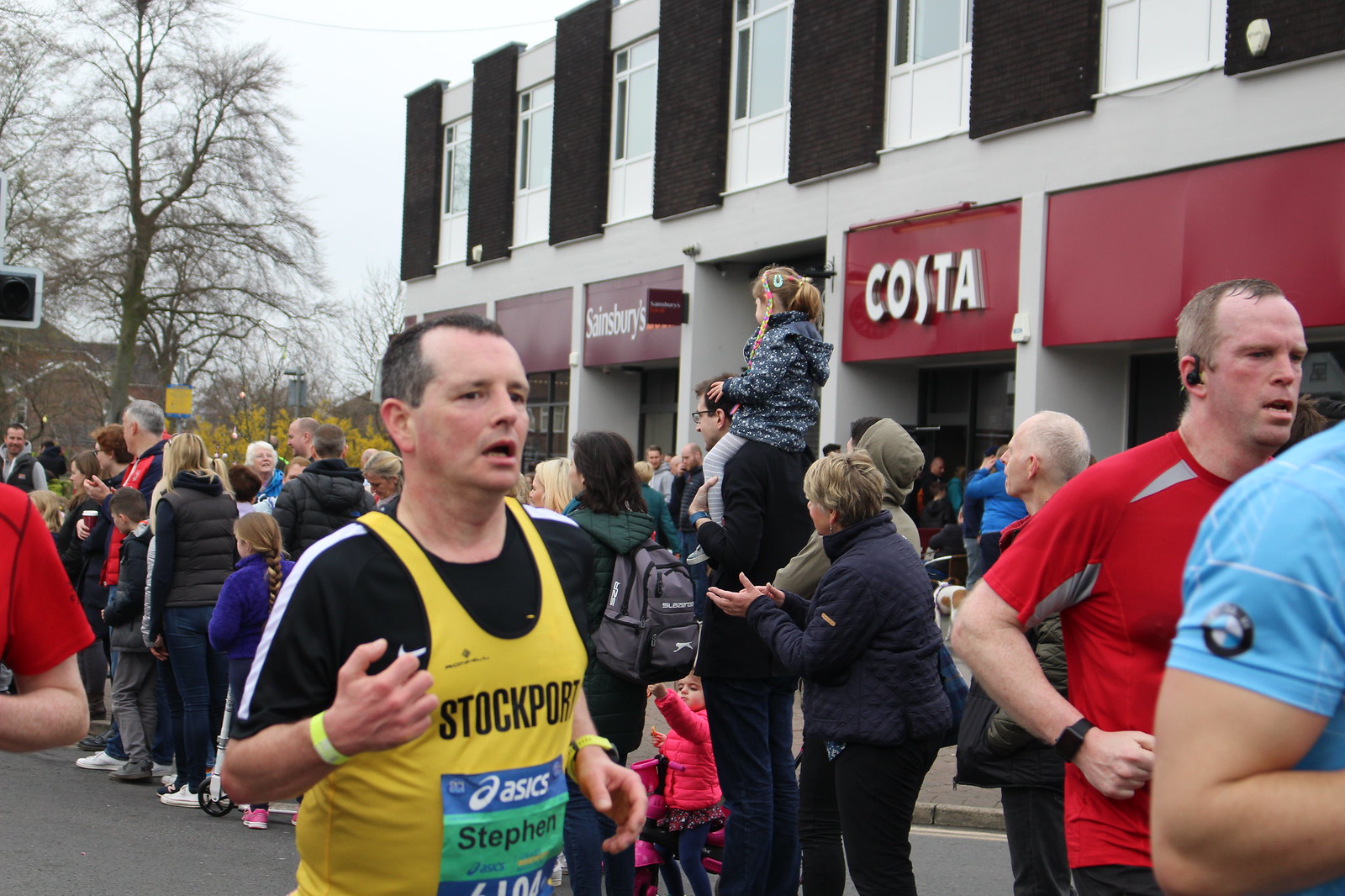In this detailed photograph of a marathon or race event, the foreground features four male runners. On the far right, only the shoulder of a participant in a blue shirt is visible, his arm poised in a running motion. Next to him on the left, a runner clad in a red shirt with a black watch is prominently displayed. Central to the image is a man in a black shirt with white stripes on the shoulders, layered with a yellow tank top that reads "Stockport," accompanied by a pinned race number. He appears tired but determined. Adjacent to him, towards the left, there's a glimpse of another runner's shoulder in red.

Behind the runners, a diverse crowd of mostly older spectators is visible, facing towards oncoming participants. Among them, a man stands out, dressed in black with glasses, hoisting a little girl on his shoulders. The background is dominated by a two-story building adorned with red signage; one sign reads "Costa" in white letters, with another indiscernible sign. Additionally, on the left, another sign appears to read "Sainsbury." The scene suggests a potentially chilly day, evidenced by spectators' jackets and a barren tree without leaves, set against a pale, wintry sky.